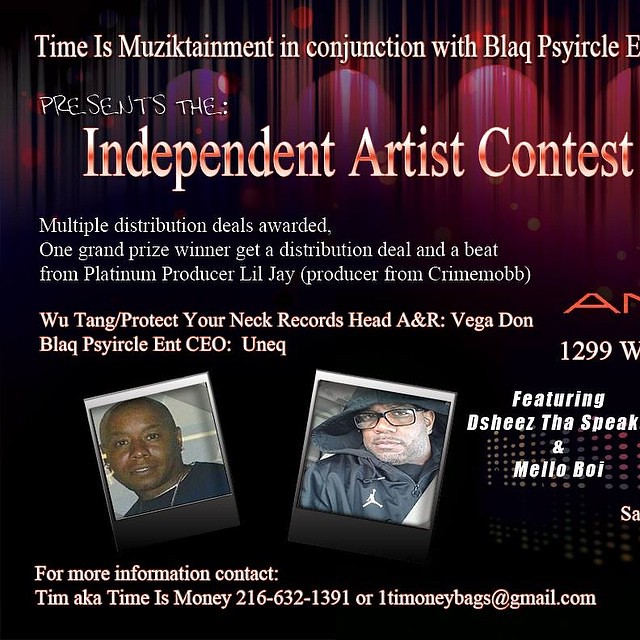A striking flyer set against an all-black background and accented with a red curtain announces: "Time is Musictainment, in conjunction with Black Pea Circle, presents the Independent Artist Contest." Prominent white and red letters underline the event's significance, promising multiple distribution deals for outstanding independent artists. The grand prize winner will receive a prestigious distribution deal alongside a custom beat from Platinum producer Lil Jay, known for his work with Crime Mob. Also featured is esteemed guest Wu Tang, Protect Your Neck Records' Head A&R, Vega Don, along with Black Circle Entertainment's CEO, Yu Nake.

Highlighted musicians Deeshee, Daspeak, and Mello Boy add to the anticipation. The flyer includes an image of two individuals: a darker-skinned man wearing a black shirt and a lighter-skinned man in a Jordan hoodie with gold accents and glasses. There are also purple dots accentuating the design. For additional information, attendees are urged to contact Tim, also known as Time is Money, at 216-632-1300 or via his email, 1tmoneybags@gmail.com.